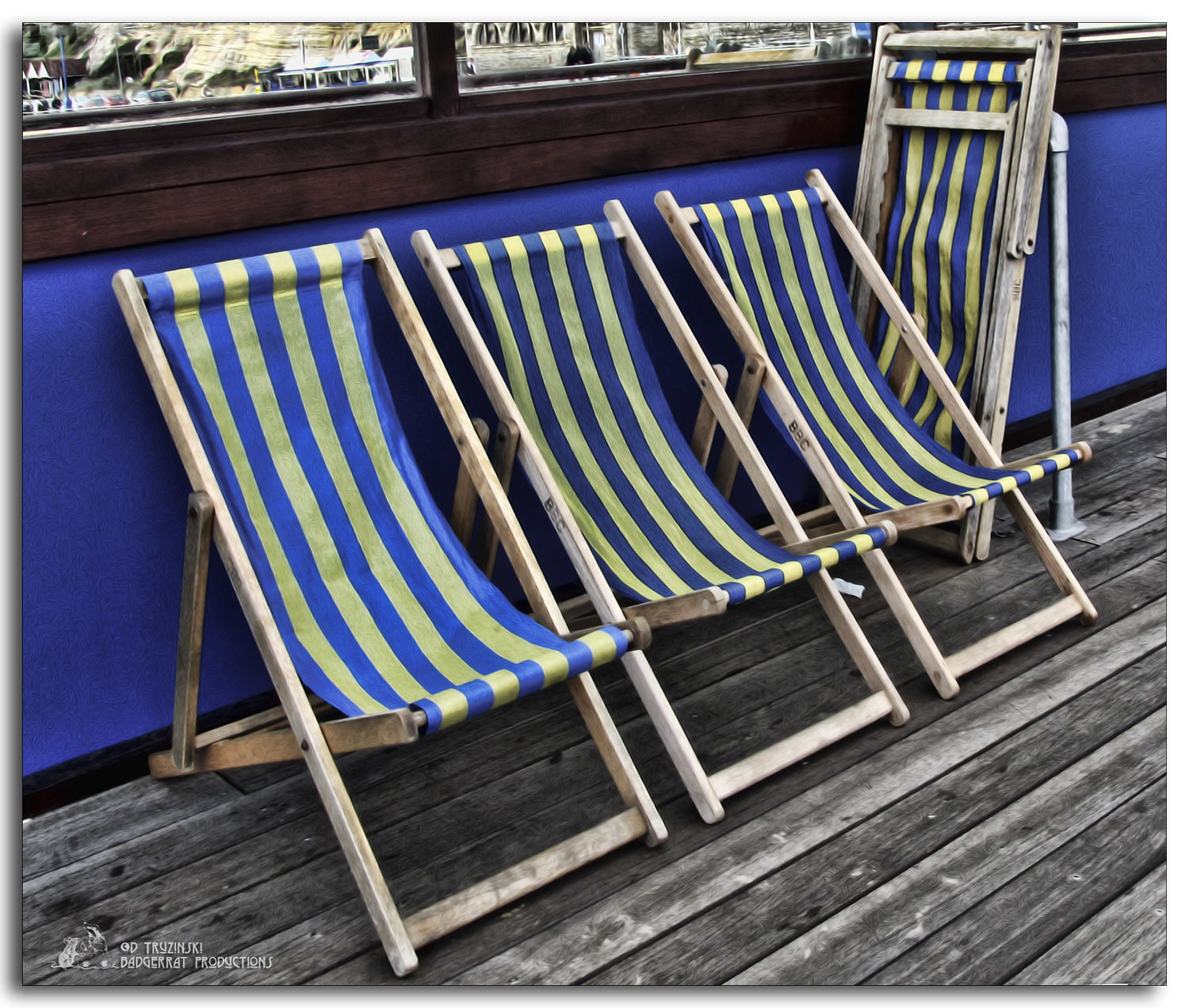In the daytime photograph, three heavily-used wooden-framed beach swing chairs, characterized by blue and yellow pinstriped fabric, are neatly arranged in a row on a weathered wooden boardwalk or dock. The chairs are constructed with a sling of cloth extending from the top of the backrest to the front of the seat, creating a free-hanging loop. A fourth chair, identical in design but folded, leans against a pipe stanchion beside the row. The backdrop of the image features a bright blue wall adorned with a dark wooden cap along the top edge. Two lower window panes set into the wall suggest a storefront, with indistinct and grainy views of boats and perhaps rocky cliffs beyond. The scene is completed by an overlay of fine white text in the lower corner, rendering it unreadable.